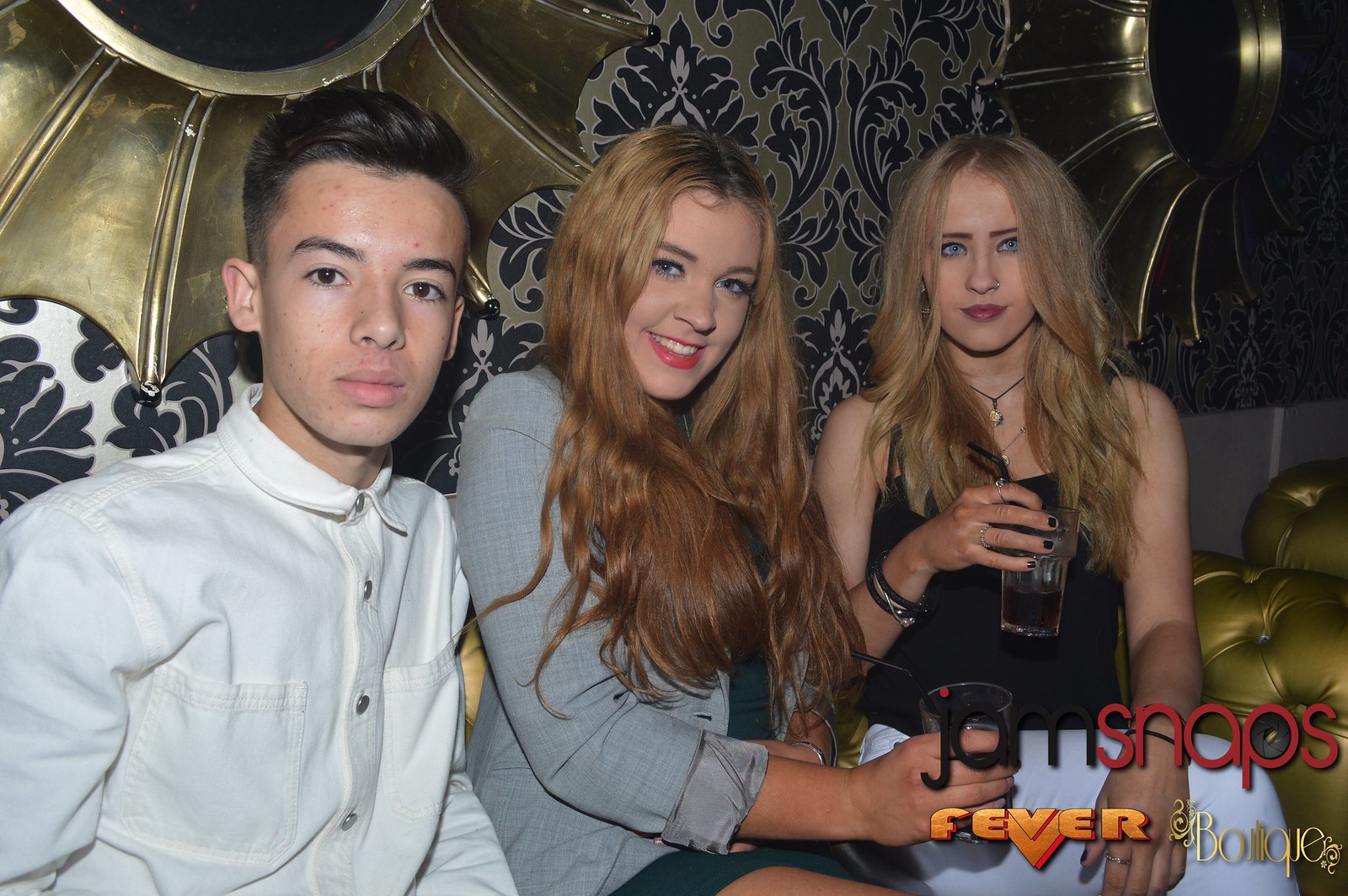In this photograph, three individuals are posing together against a lavish backdrop featuring gold wallpaper and two gilded mirrors, suggesting they could be in a bar or club, seated on a gold sofa. On the left, there's a serious-looking young male, possibly in his late teens, with short, well-groomed brown hair, wearing a white long-sleeve button-up shirt. In the middle, a smiling young woman with strikingly long, wavy red hair and dark roots, accentuated by her blue eyes and red lipstick, is dressed in a green dress paired with a gray blazer. She holds a clear cup with a straw. To her right stands another young woman, potentially the oldest, with wavy, chest-length dirty blonde hair and purplish lipstick. She is dressed in a black tank top and white pants, also holding a cup with a dark beverage and a straw. The female in the middle is the only one smiling with her teeth showing. The caption at the bottom right corner reads "Jam Snaps, Beaver Boutique." The photo captures the subjects from the waist up.